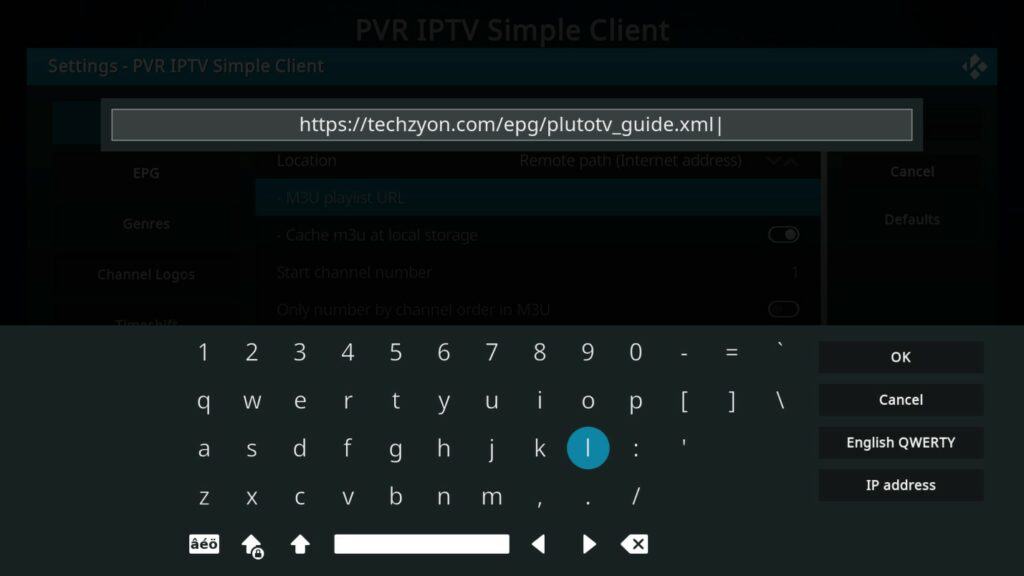This is a detailed screenshot of someone's mobile phone in landscape orientation with a predominantly black background. At the top of the screen, there is a gray search bar containing the URL "https://tegzion.com/epg/pluto-tv under sport guide.xml" in white text. The bottom part of the screen showcases an on-screen keyboard. The keyboard is gray and features a full QWERTY layout, complete with the numbers 1 through 0 aligned at the top. Specific to this keyboard, the letter "L" is highlighted with a blue circle. Below the main keyboard keys, there is a row containing various punctuation marks. The navigation features include arrow buttons pointing up, left, and right, as well as a search function. To the right side of the keyboard, the words "OK" and "Cancel" are displayed, stacked vertically. Further below, there are additional labels reading "English Priority" and "IP Address." This screenshot provides a comprehensive view of both typing and navigating functionalities available on the device.